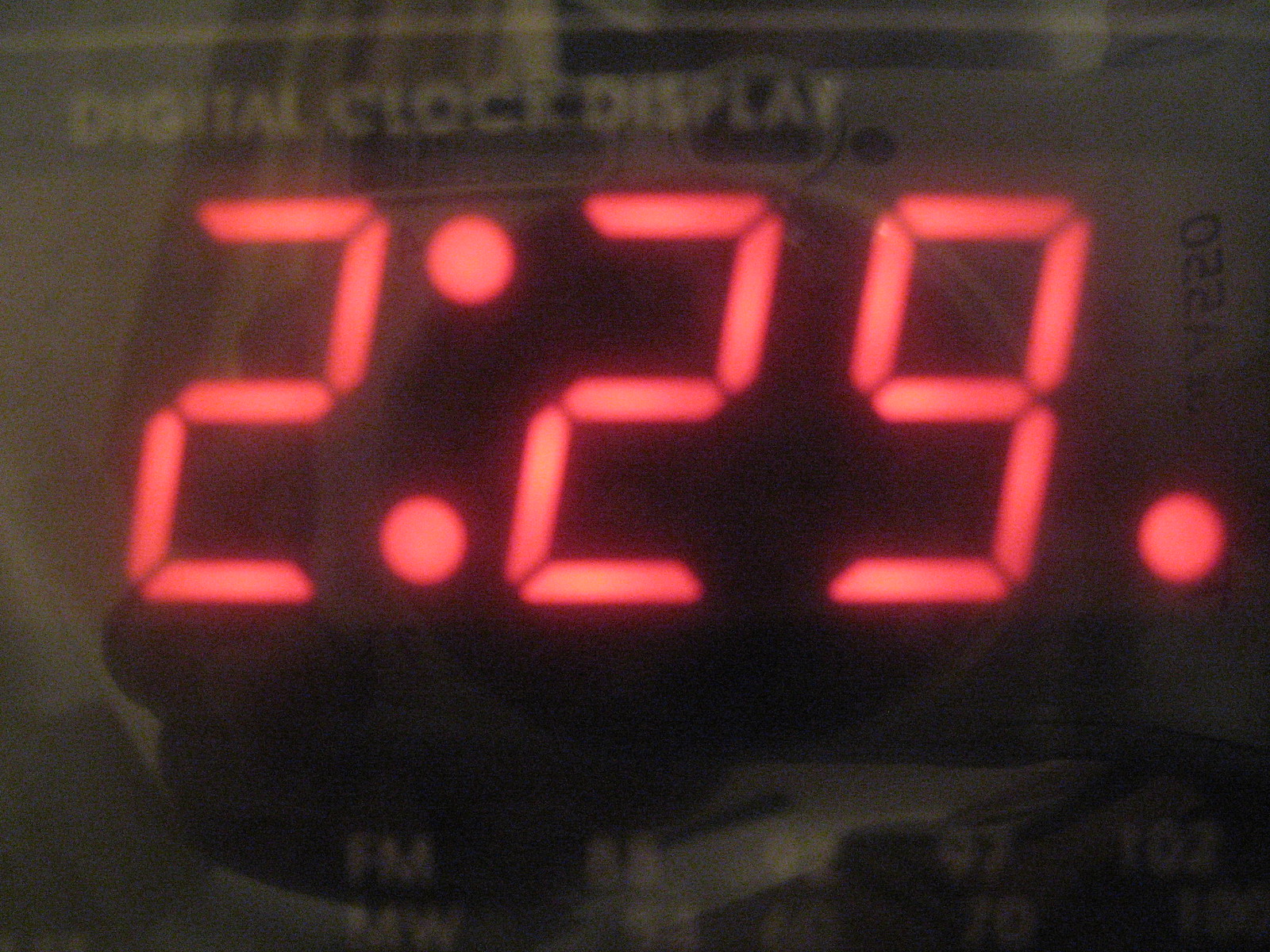The image features a digital clock display set against an all-black background. In the center of the display, the words "digital clock display" are prominently shown in white letters. The time is shown in an illuminated red, with the hour reading "02," followed by two pulsating red dots, and then the minute reading "29." To the side of the red digits, there is another small red dot. At the bottom of the display, below the clock face, there is a transparent section indicating the FM radio frequency, displaying numbers that include "88" and "97," likely indicating the radio station's range from 88.9 to 97.